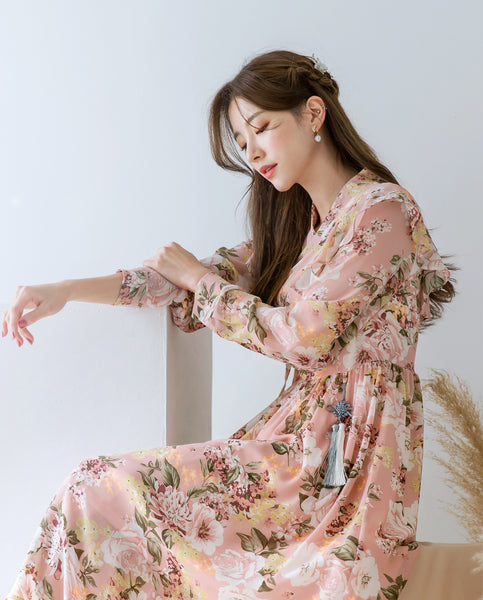This portrait-style photograph captures an Asian woman seated gracefully, seen from a side profile with her front facing left. Her right arm rests atop a staff or pole, while her left arm gently rests on her right forearm. Her hair is styled in a half ponytail, cascading over her right shoulder. She is adorned in a light pink dress, embellished with white and yellow floral patterns and accompanying leaves. She accessorizes with delicate pearl earrings and wears subtle makeup. The backdrop is a simple, light gray wall, accentuating her serene and poised presence.